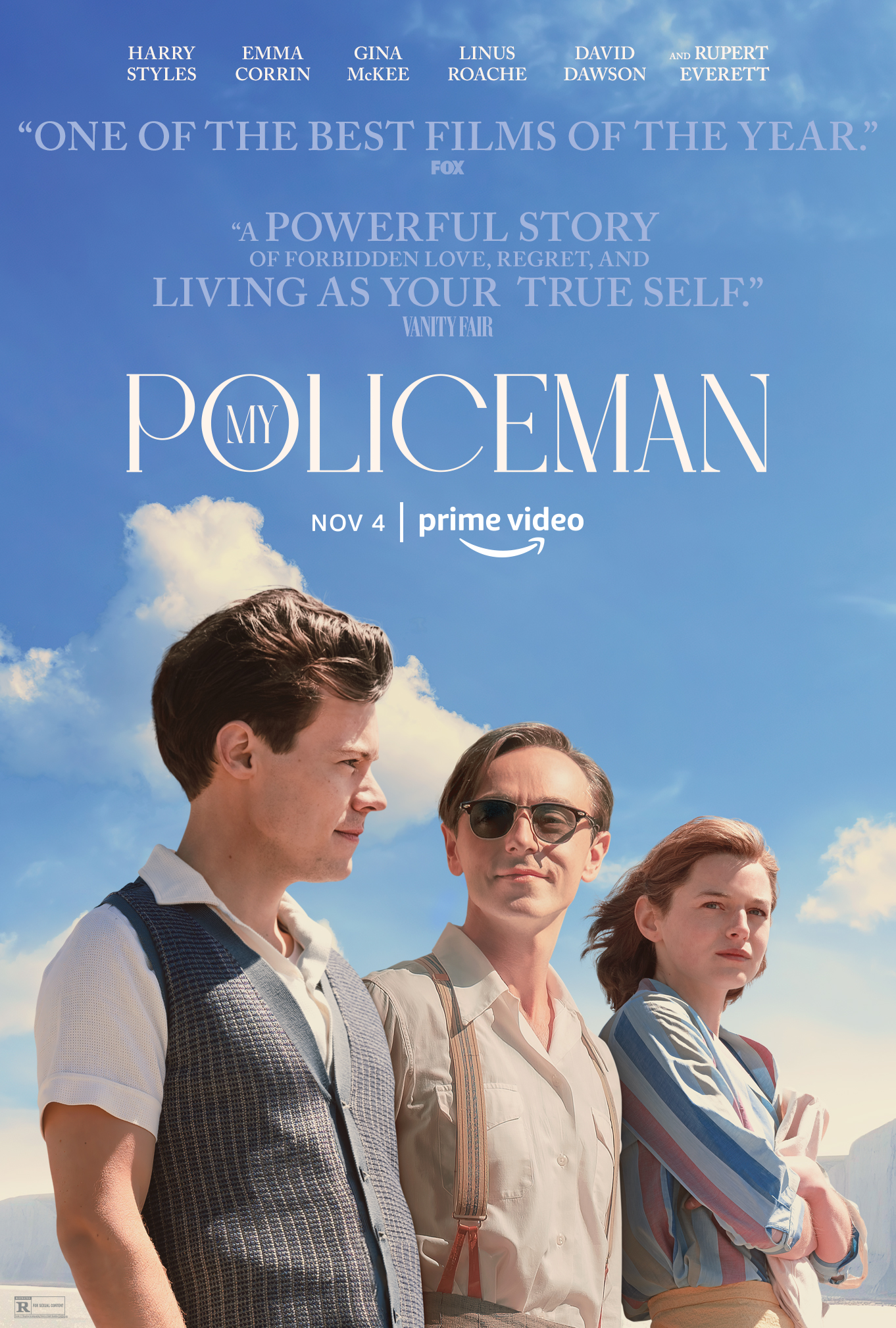This promotional poster for the Prime Video film "My Policeman" features a striking color photograph that captures a moment between three characters against a scenic background with blue skies and clouds. The poster is in portrait orientation and showcases, from left to right, Harry Styles in a white shirt with a gray vest, another male actor in a beige shirt and overall-style pants, and Emma Corrin in a light blue shirt with reddish-pink stripes and possibly beige pants or a skirt. 

The central character, played by Harry Styles, stands at the forefront looking straight ahead, while the second man gazes at him wearing sunglasses. Emma Corrin stands to the right with her light brown hair cascading softly. Above their heads, the title "My Policeman," creatively integrates the word "my" inside the letter "o" of "policeman," flanked by the release date "November 4th" and the Prime Video logo just below.

The top of the poster lists the actors' names in white font: Harry Styles, Emma Corrin, Gina McKee, Linus Roche, David Dawson, and Rupert Everett. Accompanying these are critical praises such as "One of the best films of the year" by Fox and "A powerful story of forbidden love, regret, and living as your true self" from Vanity Fair, rendered in light blue text, enhancing the elegant yet poignant aesthetic of the poster.